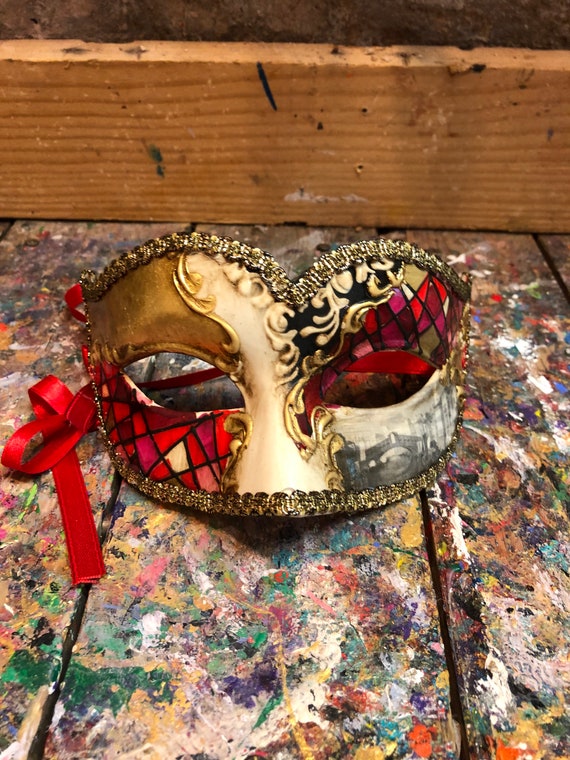This image features an elaborate Mardi Gras-style mask designed to cover the eyes and the top of the nose. The mask is adorned with intricate details, including oval eye holes with pointed ends. It boasts a rich gradient of colors: the left side transitions from dark copper to a lighter cream, with angular lines forming triangles beneath the eye that contain red, purple, and yellow sections. The right side of the mask features an etched gray cityscape at the bottom, surmounted by a yellow sky and a black background lavishly decorated with copper designs. Prominent golden fringes embellish the edges along the top and bottom, which also showcase a mix of black and copper-colored pendants. The centerpiece above the nose features a floral black and gold pattern. The mask ties around the head with a red ribbon. It's displayed on a surface resembling planks of wood splattered with various paint colors, evoking the appearance of graffiti. In the background, there is a wooden two by four with horizontal brown lines and a single black line descending from the center.